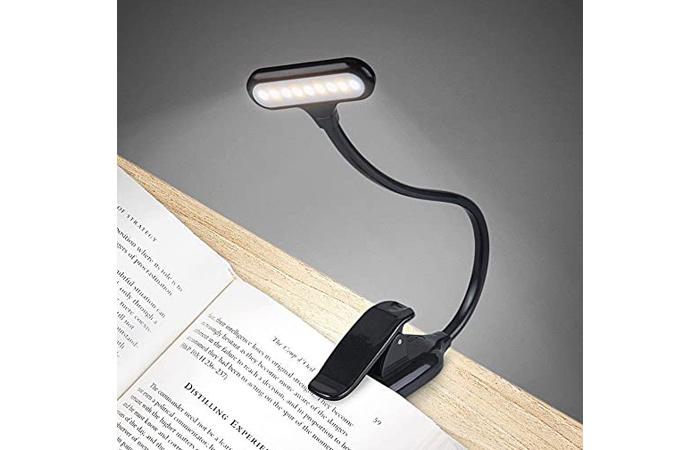The image showcases a detailed scene with a light wooden desk positioned at a 45-degree angle clockwise from a straight-on viewer's perspective. The desk holds an open book angled similarly, with visible pages. An elegant black book light with multiple small bulbs clips onto the book's right side, casting a bright white glow over the pages. The upper part of the book, including parts of the left and right pages, is visible, displaying bold text with the readable words "Distilling Experts". The background features a dark gray wall, which highlights the scene and adds contrast to the soft shadow cast by the book light. The overall impression is one of a quiet, focused space for reading or study, captured from a slightly elevated viewpoint as if the viewer is looking down at the setup.